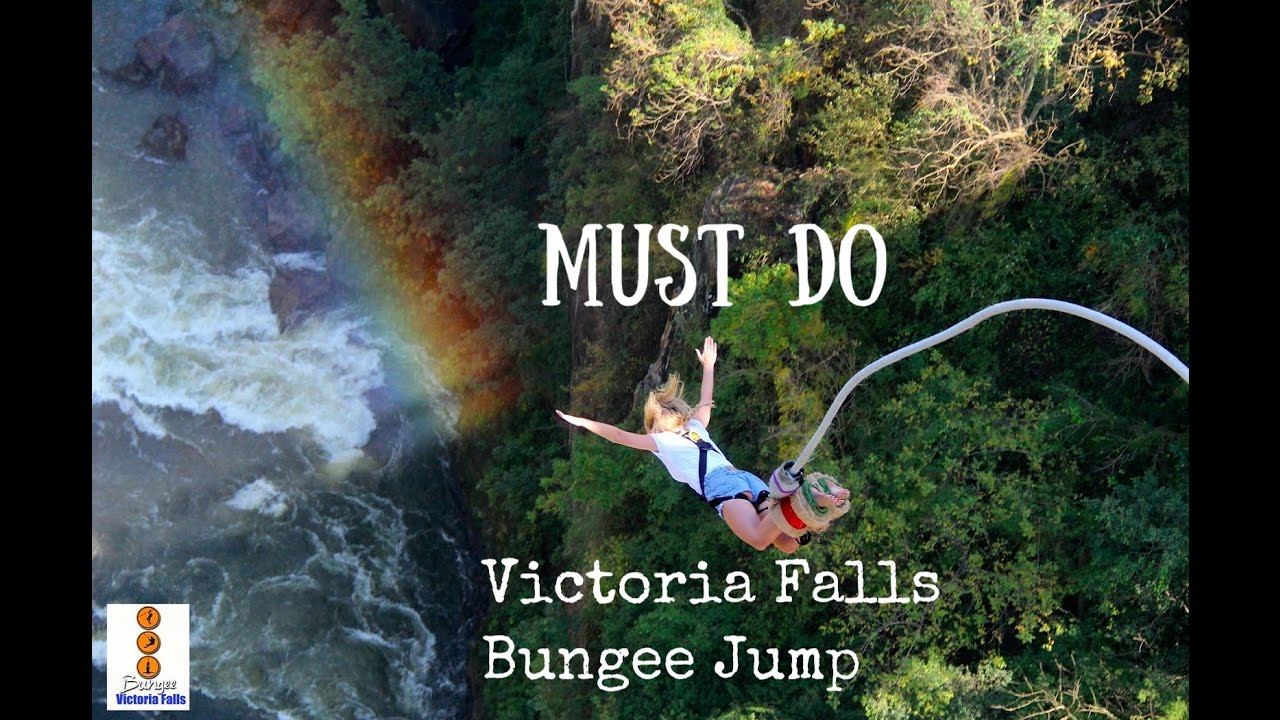The image is a full-color, rectangular photograph with its longer edge positioned horizontally, featuring an advertisement for Victoria Falls bungee jumping. The text prominently states "Must Do, Victoria Falls Bungee Jump." At the center of the scene is a person with outstretched arms, leaping into a majestic waterfall with a bungee cord securely fastened around their ankles. The daring participant, a white female with long blonde hair, is clad in a white shirt and blue shorts. 

Below her, emerald green scrub brushes frame the image, while to the left side of the scene, the expansive body of water reflects the sunlight, creating a vivid rainbow. The bungee jumper's dramatic mid-plummet position, captured against the stunning backdrop of Victoria Falls, enhances the sense of adventure and thrill. In the bottom left corner of the image, there's a logo featuring three yellow circles aligned vertically, accompanied by the words "Bungee Victoria Falls," with "Victoria Falls" in blue lettering and "Bungee" in darker text, emphasizing the exhilarating activity promoted in this visually captivating advertisement.